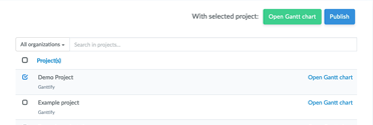This is a small, rectangular image from a website. The top and bottom edges are longer than the left and right edges. At the top portion of the image, towards the center, the text "Selected Project" is displayed in black letters. Directly to the right of this text is a green button with white letters that reads "Open Something Chart." Next to this button, there is a blue "Publish" button with the word "Publish" in white letters.

At the bottom left of the image, the text "All Organizations" is displayed with an arrow pointing downwards next to it. To the right of this, there's a search bar with the placeholder text "Search in Projects" in gray letters.

Below the search bar, there are three square checkboxes aligned vertically. The middle checkbox is filled in blue with a blue checkmark. To the right of the checkboxes, the text "Projects," "Demo Projects," and "Example Projects" are listed vertically, each with additional descriptive text written underneath them. The "Demo Projects" option is selected, causing its background to appear slightly gray.

On the right side of the image, within the gray background of the "Demo Projects" section, the text "Open Craft Projects" appears twice, written in blue letters. The space to the right of "Projects" is completely blank and white.